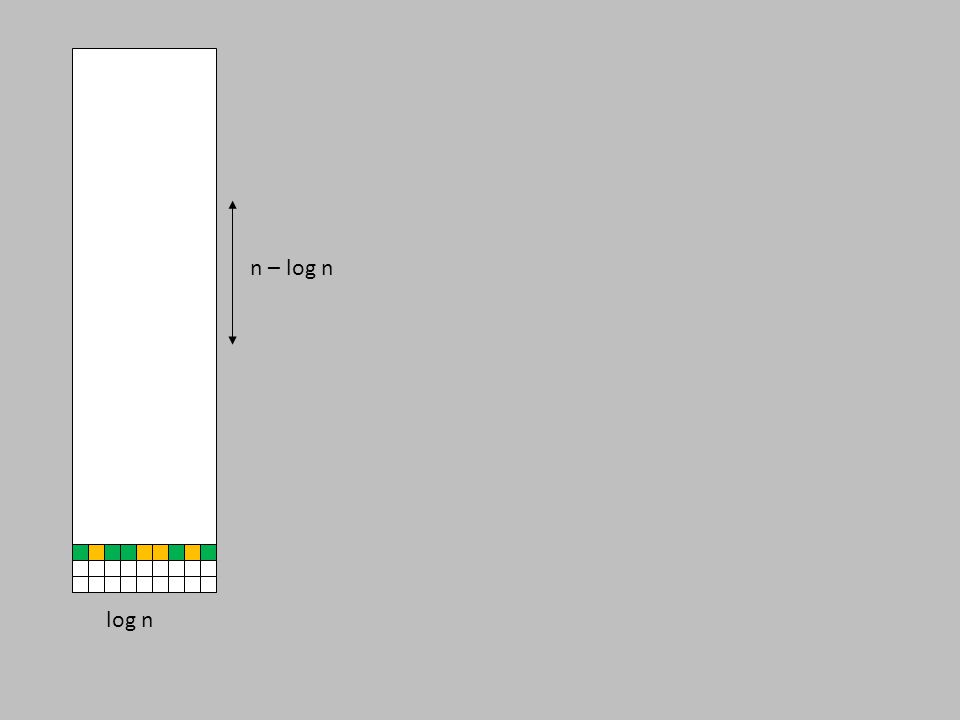The image features a gray background with a prominent vertical white rectangle on the left side. This tall rectangle is largely blank white but towards its bottom, it contains a grid of three rows consisting of ten small squares each. The bottom two rows of squares are white, while the third row alternates with squares of green and yellow following the pattern: green, yellow, green, green, yellow, yellow, green, yellow, green. Below this rectangle, the text "log n" is written in black. Adjacent to the right side of the rectangle, there is a vertical double-ended arrow marked with "n - log n."